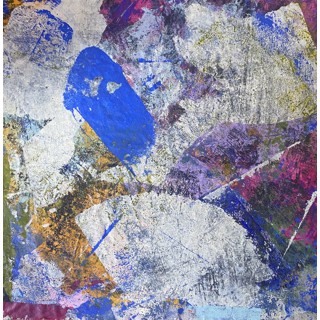This is a close-up image of a square abstract painting featuring predominantly off-white and grayish dirty white tones, interspersed with varied and vibrant brush strokes and splotches. The composition appears equidistant on all sides, characterized by a mixture of rough and coarse textures along with smoother areas. Notably, in the upper left-hand corner, there is a striking dark blue rectangular splotch surrounded by rougher white and light gray sections, accented with blue and yellow speckles. The painting also includes hints of pink and purple in this region. 

Towards the bottom right, the painting becomes more vivid, showcasing an array of colors including blue, purple, light green, and light purple, with additional rough white areas at the bottom. The top left features a vibrant blue streak, arguably the brightest color in the painting. On the right side, there are visible shades of purple, dark blue, and a pinkish hue. The bottom left corner has streaks of a dirty orange color, and at the very extreme, a horizontal line of purple that rises vertically next to a dingy yellowish-green. The top right includes another streak of dark purple. Overall, the painting is a dynamic blend of various brush strokes, lines, and splotches, with no discernable text or recognizable figures.